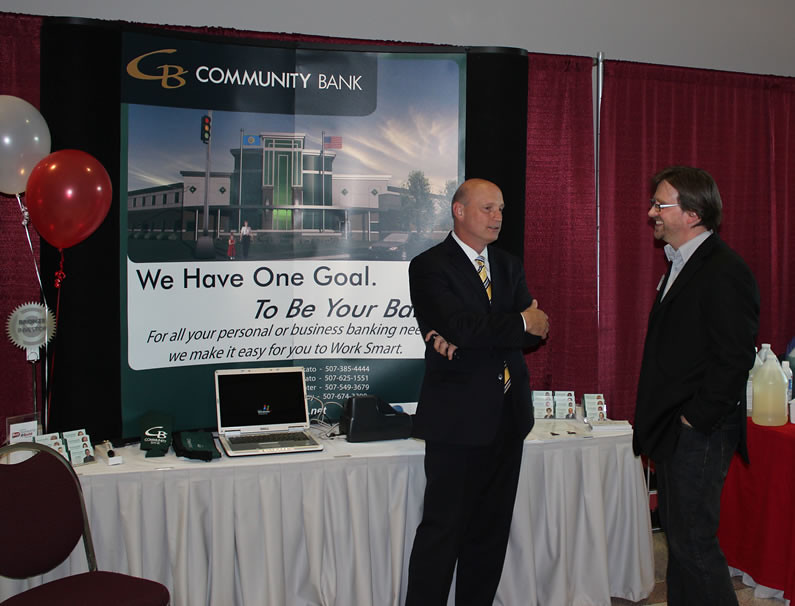This photograph, taken indoors at what appears to be a trade show or gathering, features two men engaged in conversation. Both men are dressed in black jackets that look like part of a suit. The man on the left is partially bald, wearing a full black suit with a white dress shirt and a tie featuring yellow and blue stripes. His arms are crossed over his chest. The man on the right, who has dark brown hair and glasses, is also white and is dressed in a black jacket paired with black jeans, a white dress shirt, and a black tie, with his hands in his pockets.

In the background, a table covered with a white tablecloth displays several items, including an open laptop, business cards, and promotional materials. Two balloons, one red and one white, are tied near the table. Behind the table is a large poster reading "CB Community Bank," accompanied by a photo of the bank and a motto that says, "We have only one goal: to be your bank for all your personal business banking needs. We make it easy for you to work smart." The setting is completed with a brown chair in the bottom left corner and red curtains throughout the wall, creating a formal and promotional atmosphere.